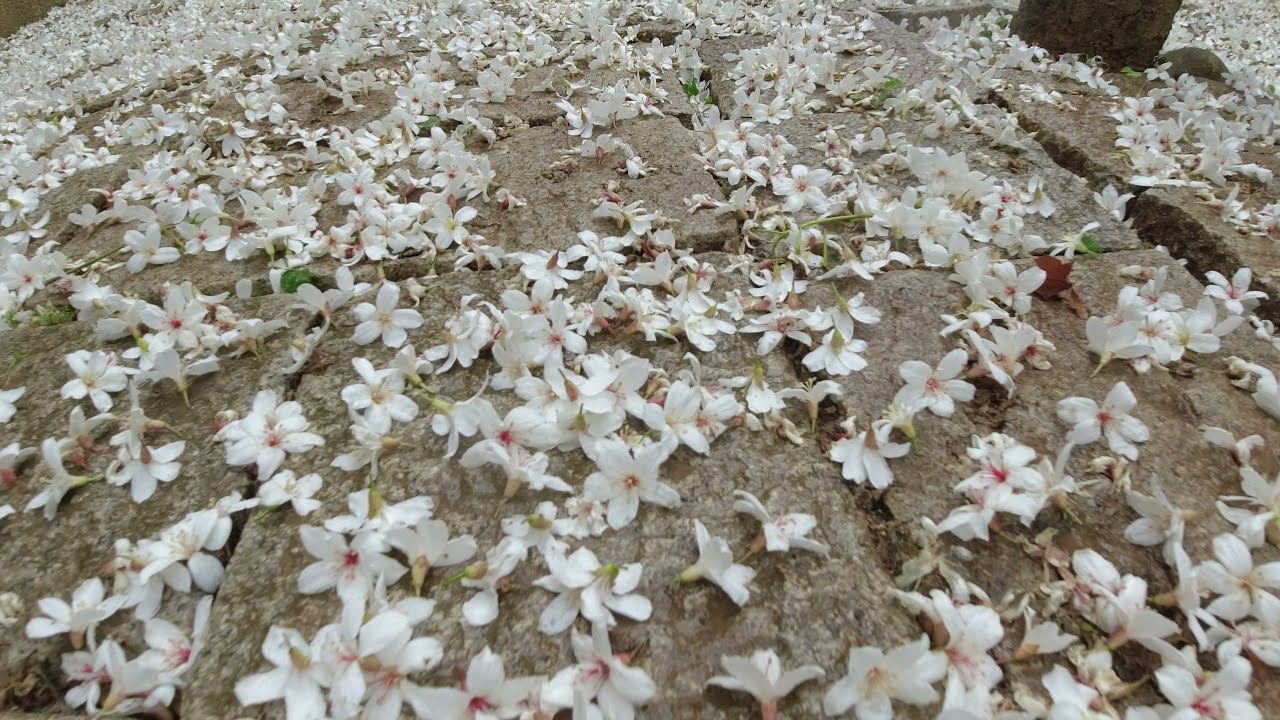The image captures a close-up view of numerous fallen white flower blossoms with five petals each, scattered densely across the ground. The flowers, which likely fell from a tree, feature blushy pink centers with reddish stamens, although a few show slight green stems or yellow hues at the core. These blossoms are sprawled over weathered, mid-toned gray-beige stone tiles, covering approximately 75% of the surface. A smattering of green grass or weeds sprouts between the gaps of the rectangular pavers. In the upper right corner, a small section of a tree trunk or post is visible, hinting at the origin of the fallen flowers, while the rest of the image is dominated by the floral overlay.